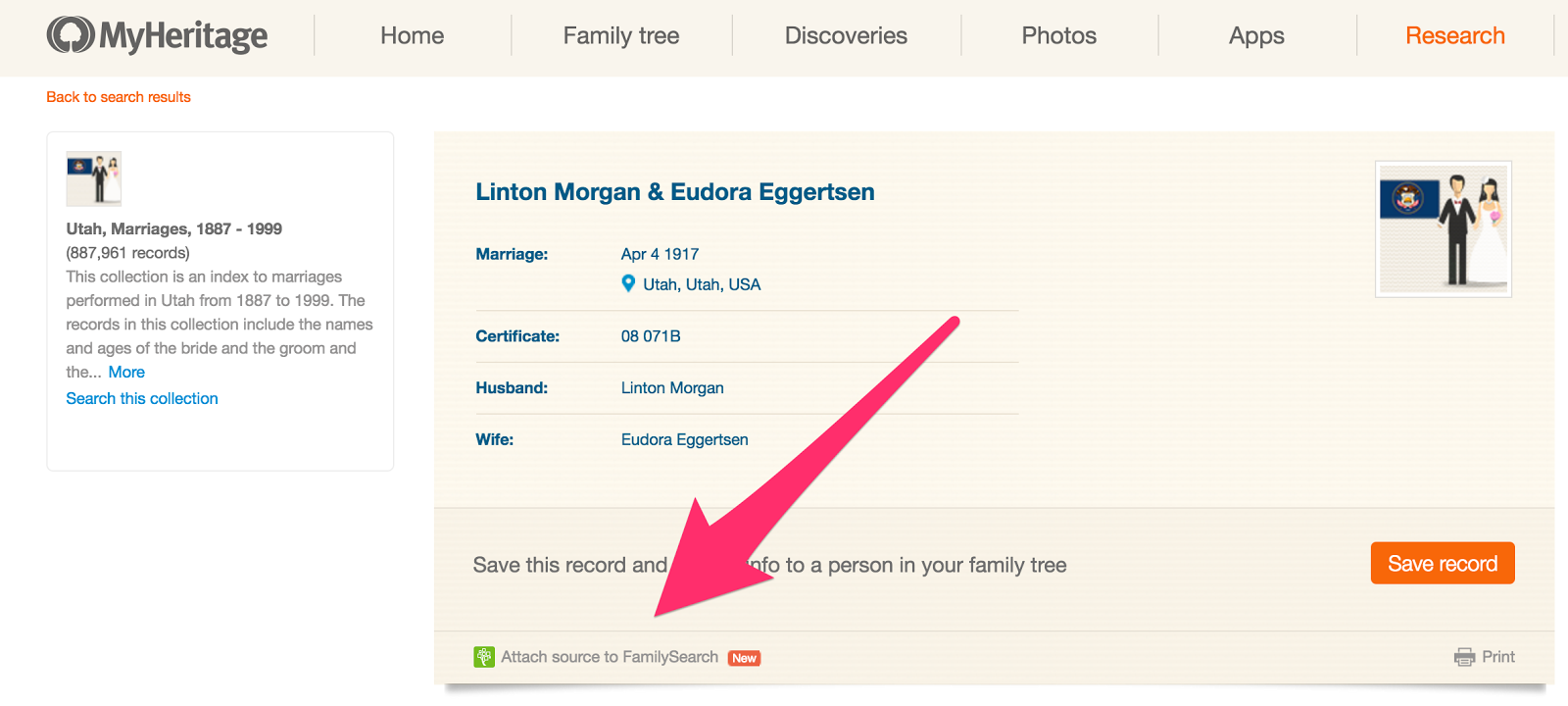This image is a cropped screenshot from the MyHeritage website, focusing on a specific section under the "Research" tab. The screenshot has been trimmed on the left, right, and bottom. On the left side of the image, there is a white background with a small box at the top left corner. This box provides information about the "Utah Marriages 1897 to 1999" collection, noting that it contains 857,961 records. The description indicates that this collection indexes marriages performed in Utah during the specified years, including details such as the names and ages of the bride and groom, followed by an ellipsis and the word "more" in blue, suggesting additional information is available.

Below this description, there is a blue link that says "Search this collection".

On the right side of the screenshot, there is a larger pink box displaying names: "Linton, Morgan and Eudora Eggertson". Further to the right, there is a smaller box with a clip art image of a bride and groom. Beneath this image, the screenshot lists details such as the date and location of the marriage, the certificate number, the husband's name, and the wife's name. 

At the very bottom left corner of the pink box, there is a blue text link that says "Attach source to FamilySearch". An edited pink arrow points directly at this link, emphasizing its significance.